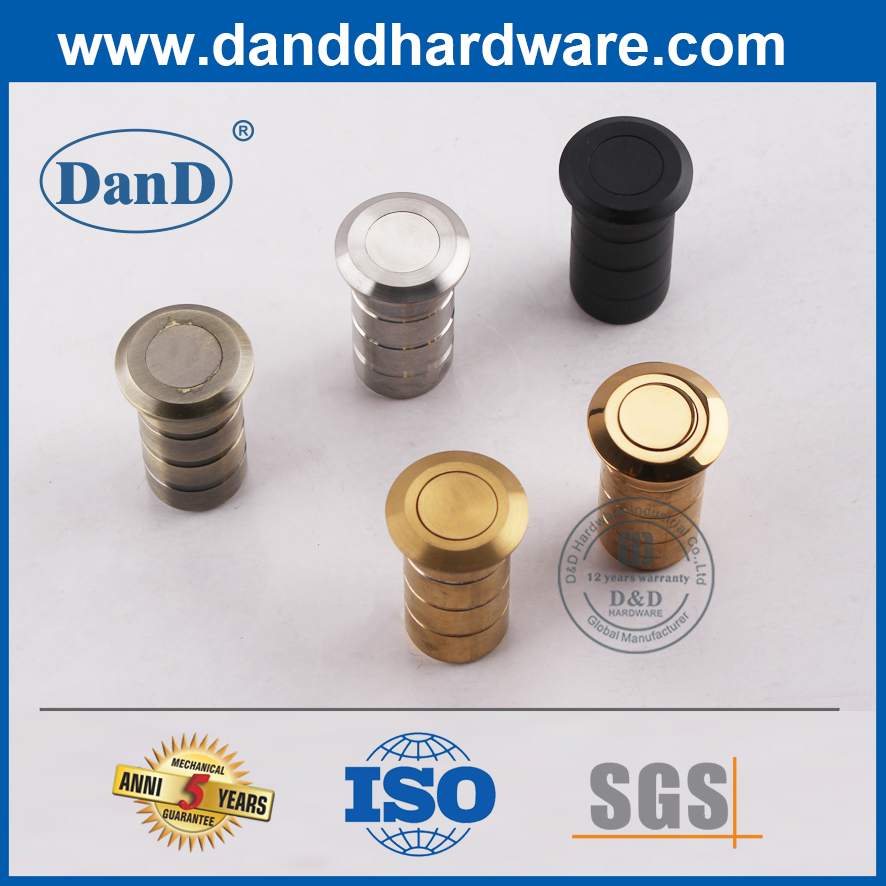The image is an advertisement from D&D Hardware, prominently featuring their logo in the top left corner. At the very top of the ad, there is a blue banner with white text reading "www.dndhardware.com," and a thin blue border surrounding the entire image. The main section showcases five different tools that resemble wide screws with flat ends. These tools are displayed in various metallic finishes, including light silver, dark black, gold, and a shinier gold, arranged in a pyramid-like formation with three in a diagonal line and two more fitting in between. At the bottom of the ad, there is a gray footer featuring awards and recognitions, including "Mechanical," "5-year Guarantee," an ISO globe symbol, and the letters "SGS" with an orange border. Additionally, a seal stamp over one of the tools states "D&D 12-Year Warranty."